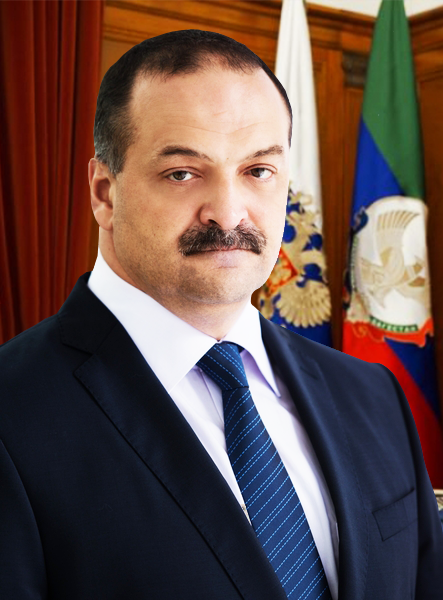In this image, we observe a man who appears to be a politician or businessman, positioned in front of a wooden-structured background, suggestive of an office or formal setting. There is a red curtain visible on the left-hand side and two flags to the right behind him. One flag features green, blue, and red stripes with a circular emblem at the center, including a bird on a white background. The other flag is primarily white and blue, adorned with a golden insignia that resembles a dragon or eagle. 

The man himself has light skin and is potentially of Middle Eastern descent. He has short, black hair that is beginning to recede, accompanied by a thick, black mustache and a subtle shaved beard. His expression is stern and serious as he gazes slightly to the left. He is dressed in a navy blue suit jacket paired with a navy blue tie featuring lighter blue diagonal stripes, and a white collared shirt underneath. The overall composition and details emphasize the formality and seriousness of the scene.